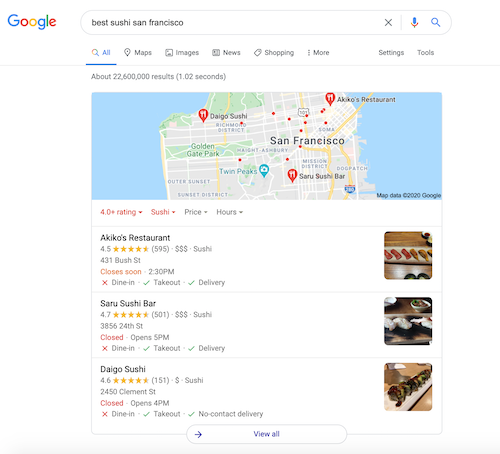The image depicts a Google search for "best sushi San Francisco." The search results are filtered to display only sushi restaurants with a rating of four stars or higher. At the top of the results page, there's a map indicating the locations of these sushi restaurants.

The first result is Akiko's Restaurant, which has a rating of 4.5 stars based on 595 reviews. It is categorized as a relatively expensive option, denoted by three dollar signs ($$$). An accompanying image shows an elegantly presented long plate of sushi, with pieces artistically arranged in a diagonal line across the rectangular plate.

The second result is Saru Sushi Bar, boasting a high rating of 4.7 stars from 501 reviewers. Like Akiko's, it is also marked by three dollar signs, signifying its place in the higher price range.

The third option is Daigo Sushi, which has a rating of 4.6 stars from 151 reviews. Unlike the previous two, Daigo Sushi is noted for its affordability, indicated by a single dollar sign ($), making it the most budget-friendly choice among the top results.